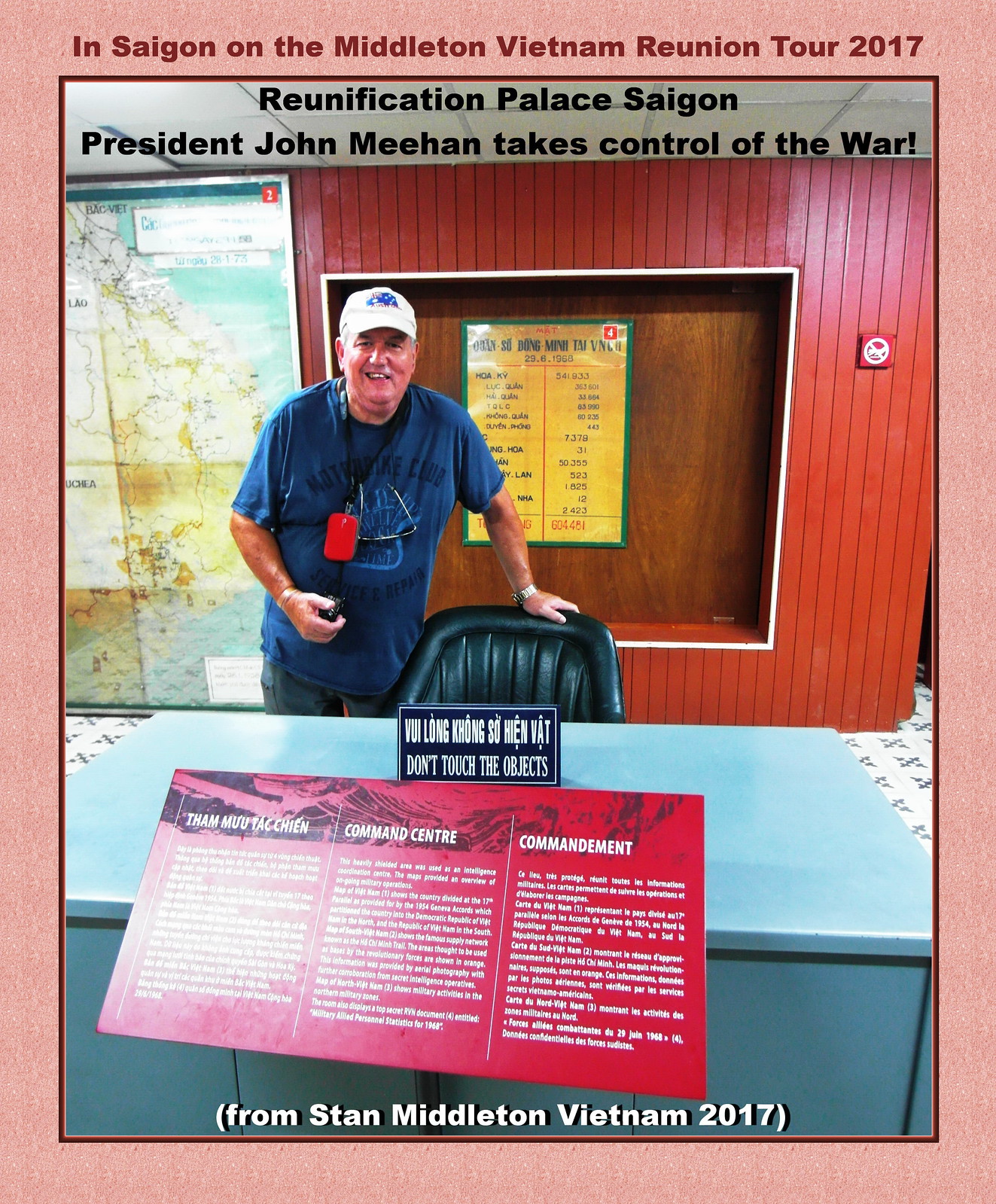In this picture, taken during the Middleton Vietnam Reunion Tour 2017, we see an elderly man posing in front of what appears to be an exhibit at the Reunification Palace in Saigon. He stands behind a small table, to the left of a black leather chair, with his hand resting on it, despite a sign that reads in both Vietnamese and English, "do not touch the objects." The man is wearing a white hat and a red tag around his neck. A map is displayed on the wall next to him, and there is a yellow and red plaque detailing the command center behind him. At the top of the image, there's text that reads, "In Saigon, on the Middleton Vietnam Reunion Tour 2017, Reunification Palace, Saigon, President John Meehan takes control of the war." At the bottom, it says, "From Stan Middleton Vietnam 2017." This photo captures a poignant moment of a veteran revisiting a significant historical site where he once served, reflecting on past events and his involvement in the war.